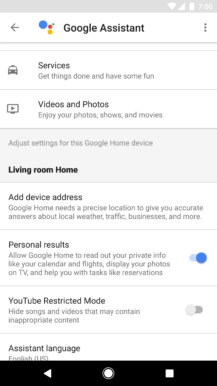Screenshot of a smartphone displaying Google Assistant settings. The interface features various service categories including a section with an icon resembling a taxi cab, titled "Get things done and have some fun." Directly below, there is a section labeled "Videos and photos" which suggests options for enjoying photos, shows, and movies. A gray box follows, prompting the user to "Adjust settings for this Google Home device," with a bold header stating "Living Room Home." Beneath this, instructions to "Add device address" highlight the importance of providing a precise location for accurate local information such as weather, traffic, and business queries. The next setting, "Personal results," is enabled (indicated by a blue dot), allowing Google Home to access private information like calendar events and flight details, and to display photos on a TV, as well as assist with tasks such as reservations. The "YouTube restricted mode" is currently turned off, which would otherwise hide content deemed inappropriate. The final section specifies the "Assistant language" set to "English (US)."